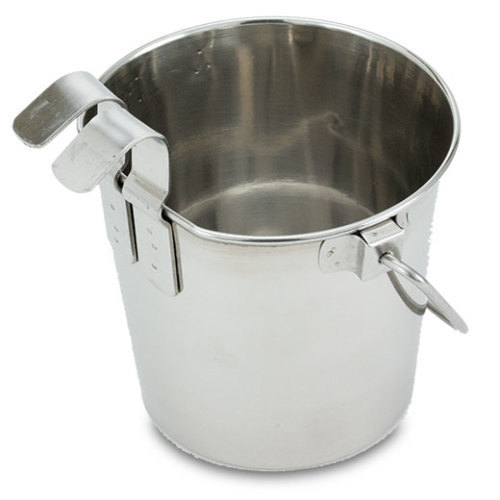A highly reflective, silvery-gray stainless steel bucket is positioned centrally against a clean, solid white background, typical of a professional studio setting. The bucket's round mouth is interrupted by a slightly flattened section where two metal hooks are securely welded to the exterior. These hooks, identical in color and material to the bucket, suggest possible uses for attaching or hanging. A sturdy handle, also made of metal, arcs from the right side of the bucket, though it rests in a down position. Slight shadowing beneath the bucket adds depth to the stark white surface. The smooth, shiny finish of the bucket emphasizes its polished, metallic construction, suitable for various practical applications.